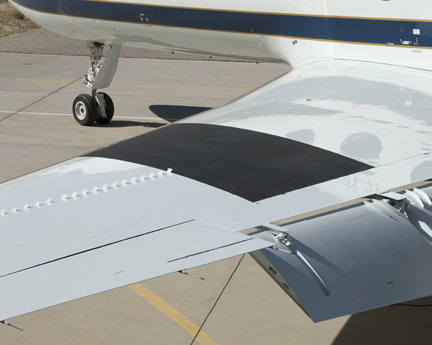The color photograph, taken in landscape orientation, captures a close-up view of an airplane on the tarmac. The focus is predominantly on the airplane's wing, which extends diagonally from the bottom left to the top right of the image, converging with the white fuselage adorned with a blue horizontal stripe. The wing itself features a prominent black rectangle in the center and flaps in a down position, revealing a dark gray hue. The front landing gear is visible in the background, indicating that the aircraft is parked. White runway lines and a faint yellow line are discernible on the clean and smooth gray pavement. Shadows beneath the plane and on the wing add depth to the image, enhancing its realistic and well-maintained appearance. The photograph appears to be taken from a slightly elevated angle, possibly from a drone or a high vantage point, offering a detailed and comprehensive view of the aircraft wing and part of its body.